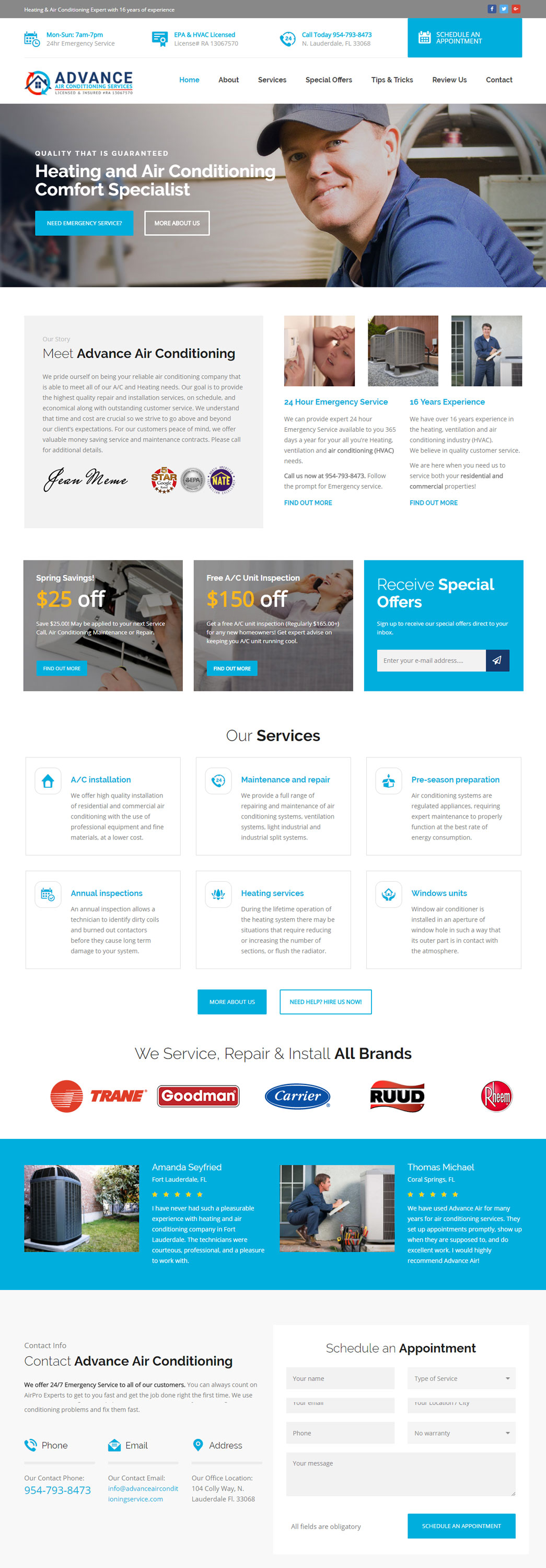Here's a cleaned-up and detailed descriptive caption for the image of the website:

---

The image displays a comprehensive view of a website belonging to a company named "Advanced Air Conditioning." At the top of the page, partially visible text likely references the company's name. Prominently featured is a photograph of a gentleman wearing a hat and a blue shirt, smiling warmly in front of a house. To the left of his image, white text states "Heating and Air Conditioning Comfort Specialist."

Below the image, a gray box contains the message "Meet Advanced Air Conditioning," along with a personal message and a signature in the bottom left corner. Scattered within this section are various smaller images, including an air conditioning unit, a person with their hand on their head, and another individual in a blue shirt holding an object.

Moving further down, promotional offers are highlighted with images displaying "$25 off" and "$150 off." Adjacent to these offers is a blue box prompting users to "Receive Special Offers," complete with a white text field for user input. Below, the section titled "Our Services" includes several smaller text boxes detailing the range of services offered by the company.

Further down, a statement declares, "We service, repair, and install all brands," alongside logos of notable brands such as Trane, Goodman, Carrier, and Ruud.

At the bottom of the page, a blue text box showcases two images: one of an air conditioning unit and another of a man inspecting a unit. The footer includes options to "Schedule an Appointment" and "Contact Advanced Air Conditioning."